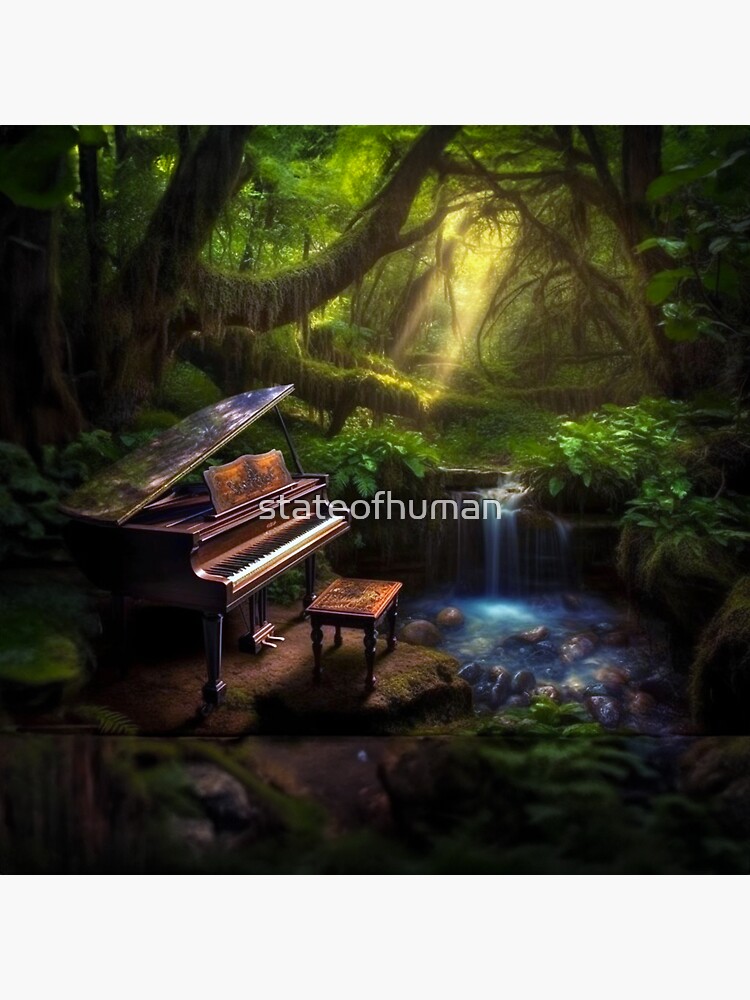This highly realistic illustration, reminiscent of AI-generated art, features an old, dark brown grand piano situated in the left foreground of a dense forest. The piano's lid is propped open, revealing its bright white keys, while its slightly dirty, aged surface hints at a burnt orange hue. A square-shaped bench, matching the piano's color, stands in front of it, with dark black engraved legs. 

In the backdrop, a thick forest brimming with various trees, hanging vines, and limbs intertwines, creating a rich tapestry of greenery in shades from dark brown to bright green. Sunlight streams through a gap in the canopy in the upper right, illuminating parts of the scene. Just to the right of the piano, a small waterfall cascades over numerous rocks into a stream, adding a serene aquatic element. 

The image also contains the words "state of human" in white, serving as a watermark.